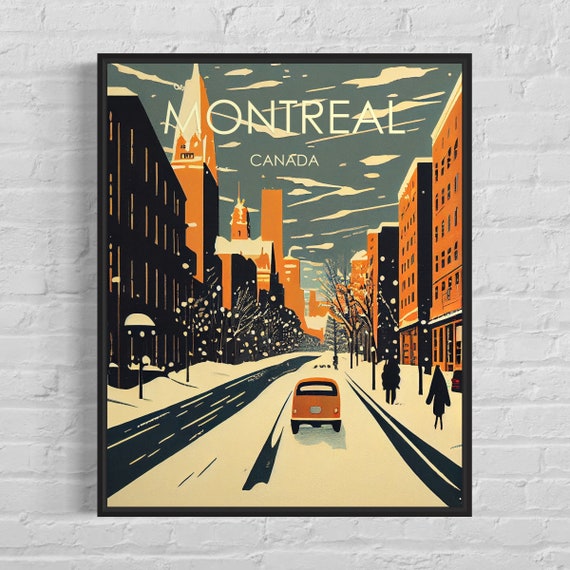This framed poster, professionally photographed and artistically composed, is affixed to a white painted brick wall. The black-framed artwork advertises Montreal, Canada, with "Montreal" displayed prominently in large white text above "Canada" in smaller, all-capital letters. The scene depicts a snowy urban street. A brownish-orange car or van is driving away from the viewer along a partially visible gray road, with its shadow cast on the snow. Two pedestrians, represented as black silhouettes, walk on the snow-covered sidewalk beside the vehicle. Lining the street are various detailed buildings: a black building on the left, several high orange towers on the right, and a few rectangular, tannish, possibly brick structures. Trees are visible along the street, adding to the intricate and inviting winter cityscape.